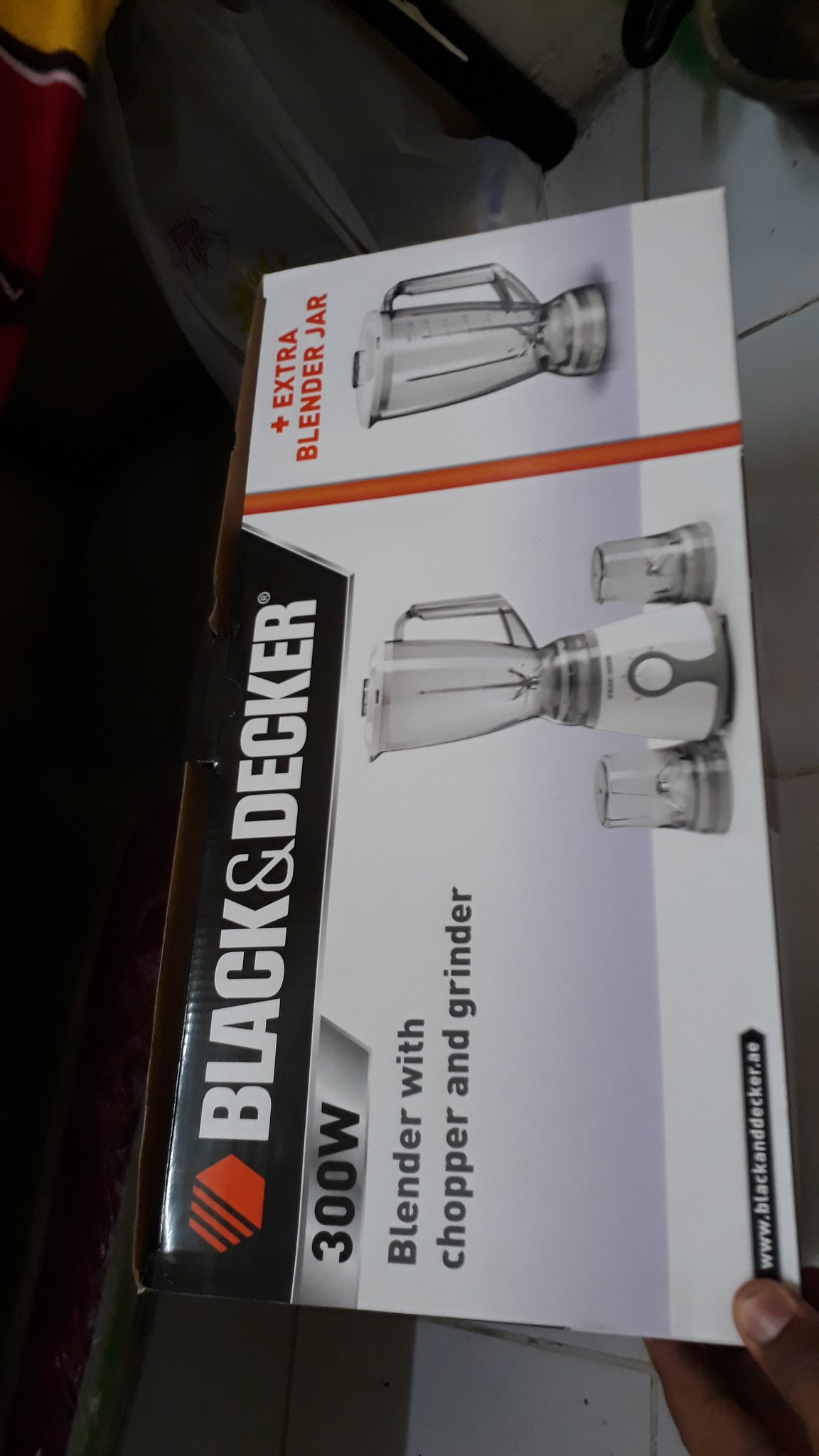The image depicts a box for a Black & Decker 300W Blender with Chopper and Grinder, held vertically by a black male hand visible in the bottom right-hand corner. The dark left side of the image contrasts with the lighter, well-lit right side, possibly indicating the background. The box itself is horizontally oriented with a prominent Black & Decker logo in orange, featuring white lettering on black bands near the upper edge. The box showcases images of the blender with its chopper and grinder attachments on either side, along with an extra blender jar highlighted by an orange stripe. Near the thumb, the box faintly displays the Black & Decker website, possibly www.blackanddecker.com. The overall presentation suggests the need for the image to be rotated clockwise to be viewed correctly.